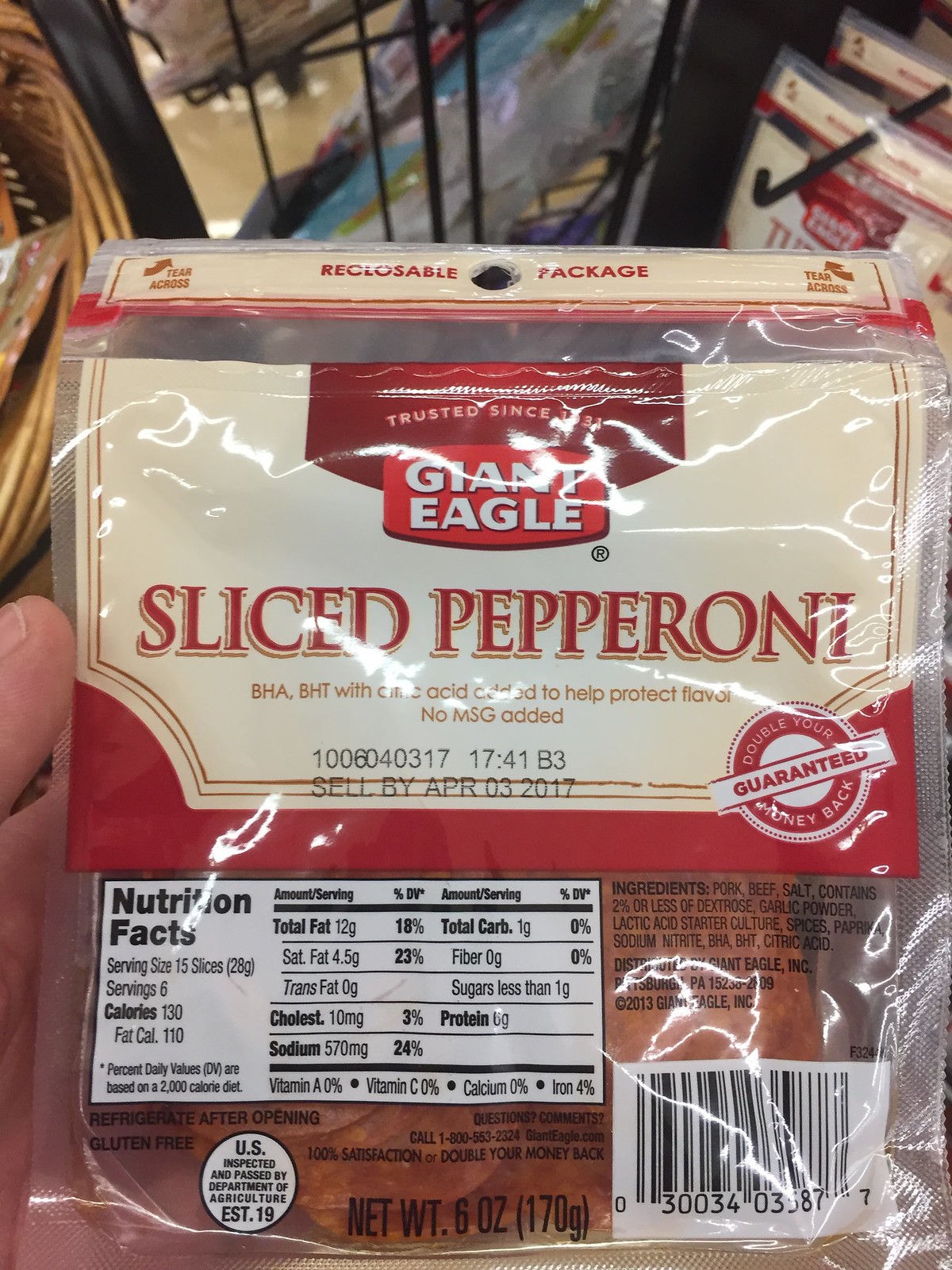In this photograph, a person's thumb is visible as they hold a six-ounce package of sliced pepperoni from the Giant Eagle brand. The packaging features a color scheme of tan, off-white, white, red, and black. The front of the package displays a U.S. inspection seal and a black-and-white barcode. Despite the light reflection on the package, the detailed nutrition facts label remains readable. The serving size is noted as 15 slices, with 6 servings per container. Each serving contains 130 calories, with 12 grams of total fat, 4.5 grams of saturated fat, and no trans fat. The cholesterol content is 10 milligrams, while sodium is 570 milligrams. The package also documents 1 gram of total carbohydrates, 0 grams of dietary fiber, and less than 1 gram of sugars. Although there is a light glare partially obscuring the protein information, other details indicate 0% of vitamin A, 0% of vitamin C, 0% of calcium, and 4% of iron per serving. In the background, additional packages of products and a metal black hanger are slightly visible, adding context to the setting of the photograph.